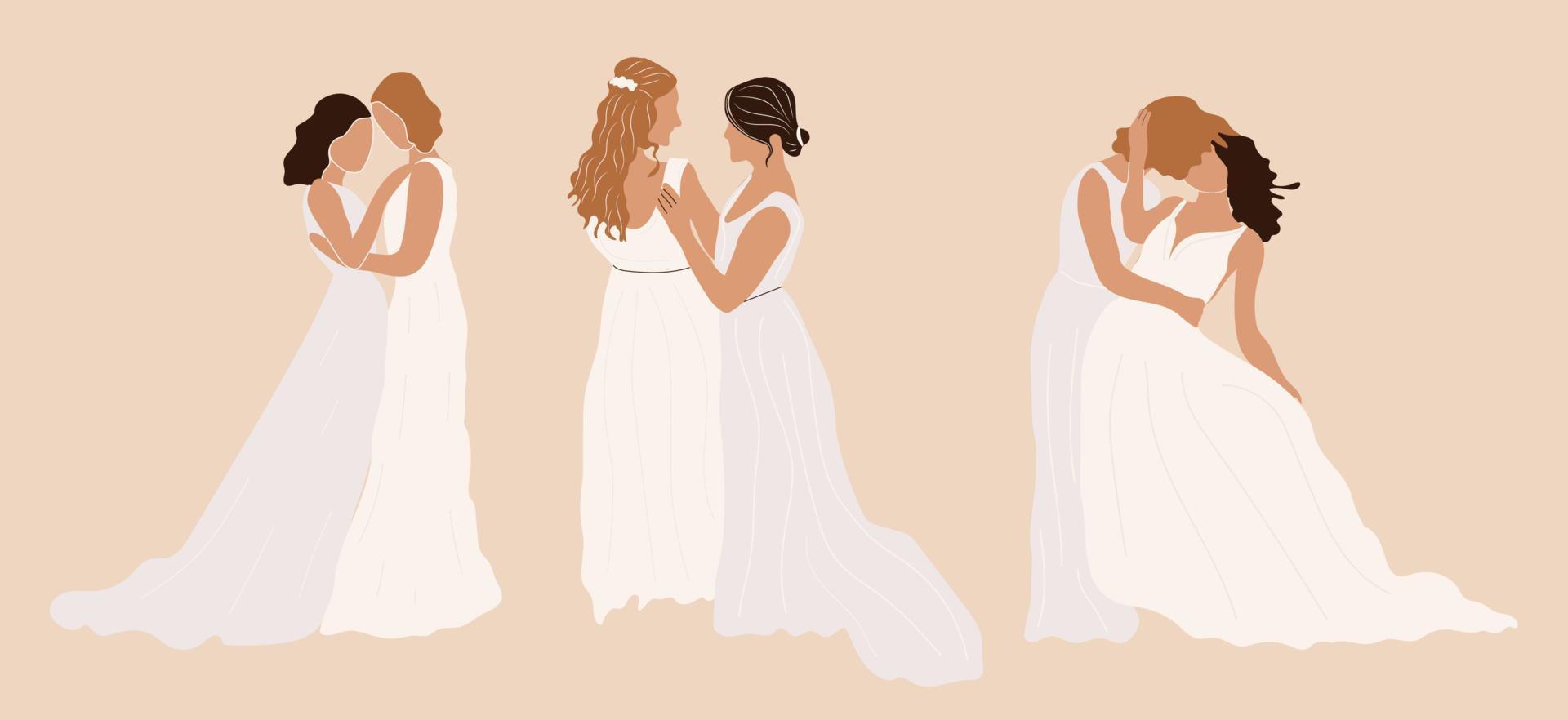This graphic image, set against a cream-pink background, depicts three distinct lesbian couples arranged in a horizontal landscape layout. Each couple consists of women clad in long, sleeveless dresses, with the attire of each pair comprising both white and off-white (or mildly gray) shades. The facial features are absent, providing a minimalistic style without eyes, noses, or mouths, and the skin tones of the figures suggest a Caucasian tone.

On the left, the couple is portrayed in an intimate embrace. The woman on the left, with black hair, wears a long off-white dress that trails to the floor. She holds the shoulder of her partner, a brunette with short brown hair in a white dress. Their foreheads gently touch, conveying a sense of closeness and affection.

The middle couple features a woman with long brown wavy hair wearing a white dress. She is positioned on the left, turned away from the viewer, while her partner with black hair tied in a bun stands on the right in an off-white dress. They appear connected and engaged with each other, emphasizing their bond.

The couple on the right is depicted in a dynamic pose suggestive of dancing or a deeply affectionate moment. The woman on the left, with short brown hair and dressed in white, holds her partner, who is leaning back with short wavy black hair and wearing an off-white dress. They are engaged in a passionate kiss, emphasizing their intimate connection.

The overall scene is versatile in setting, potentially interpreted as either outdoors or indoors, with minimalistic yet detailed elements emphasizing the romantic and affectionate nature of each couple.